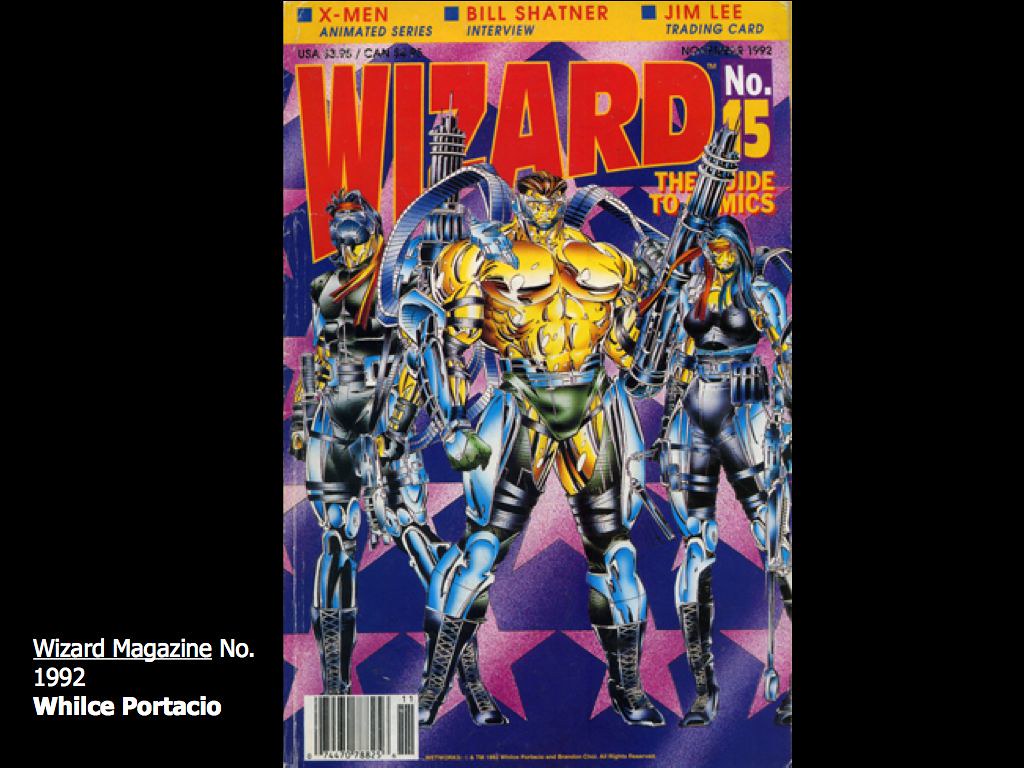The image is a detailed cover page of "Wizard Magazine" issue number 15, dated November 1992. The background of the cover is predominantly black, with a diagonal strip of purple adorned with pink stars. On the bottom left corner, there's text in white font that reads "Wizard Magazine NO.1992 Will Sportaccio" and a barcode with the numbers 74470 78825.

Dominating the center of the cover, there are three comic-book characters who appear to be warriors clad in metallic armor. The central figure is a male dressed in a golden armor suit on top, blue and silver armor pants, wearing a mask, and has tentacles emerging from his body. He's holding a futuristic gun. Flanking him are two female warriors in similar, robotic-style armor outfits, their attire made from metal and steel, enhancing their robotic appearance. 

At the very top of the cover, there's a yellow banner featuring three bullet points: "X-Men Animated Series," "Bill Shatner Interview," and "Jim Lee Trading Card." The main title, "Wizard," is emblazoned in bright red font with a yellow outline. Adjacent to the title are the words "No. 15" with the "No." in white and the number "15" in yellow. The pricing is listed below: "USA $3.95 Canada $2.95." Additional unreadable text is obscured by the central illustration.

Overall, the cover combines a striking color scheme with iconic comic-book themes and detailed character illustrations, encapsulating the essence of a vibrant, early '90s comic book.